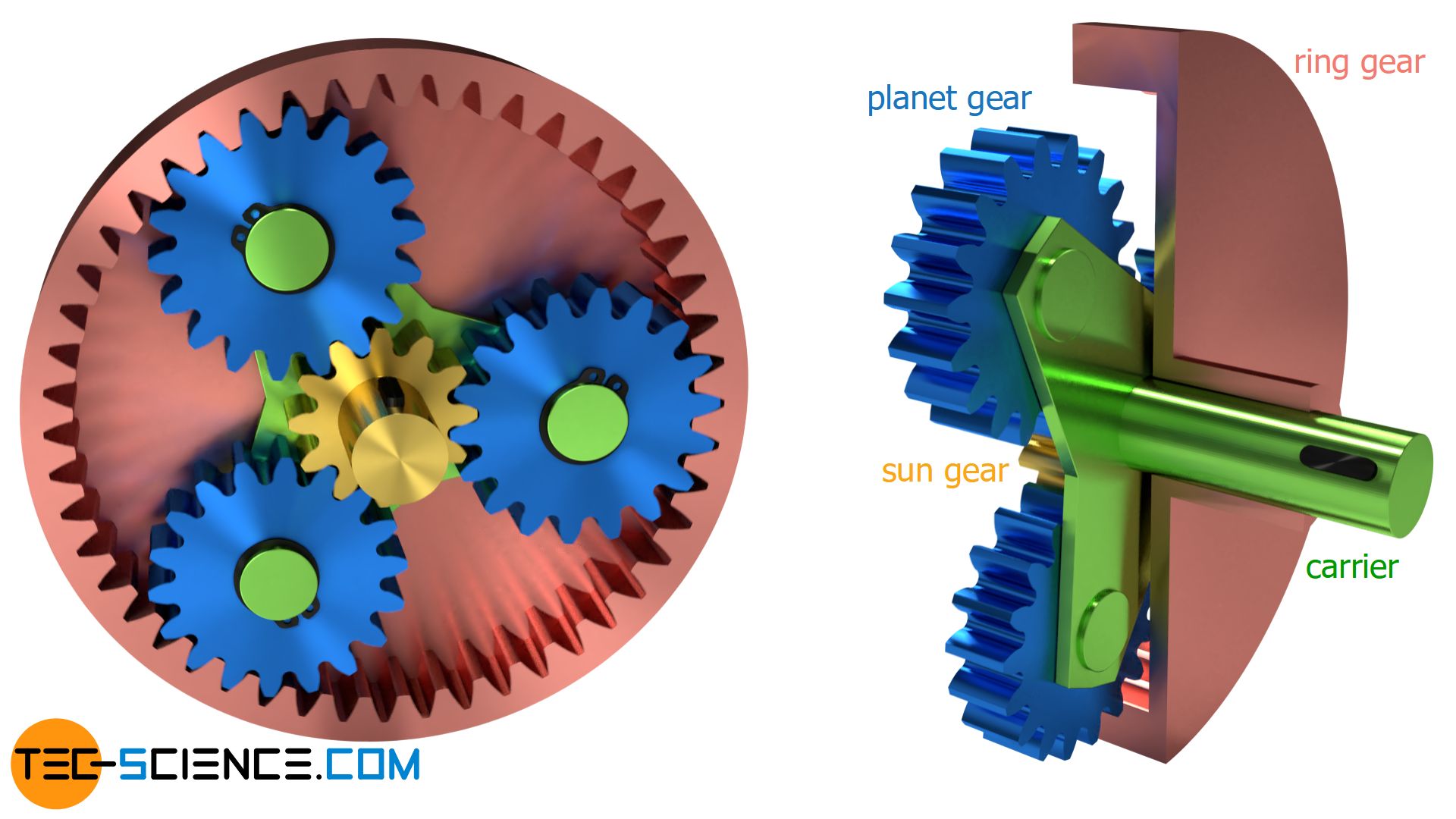This detailed color illustration from TechScience.com, identifiable by its logo in the bottom left corner, stands out against its white background. On the left side, a coral-colored, rust-like ring gear forms the outer boundary of a round wheel, with evenly spaced notches along its inner edge. Within this ring are three symmetrical blue planet gears, each featuring green centers. At the heart of the arrangement lies a centrally positioned gold sun gear. 

The right side provides a technical cross-section of the gear system, meticulously labeling each component: the coral ring gear on the perimeter, the blue planet gears nested within, the central gold sun gear, and the green carrier which aligns through the cores of the blue gears. The diagram's attention to detail, combined with the clear, crisp colors, gives the gears a shiny, metallic appearance, conveying both their aesthetic appeal and functional intricacies.